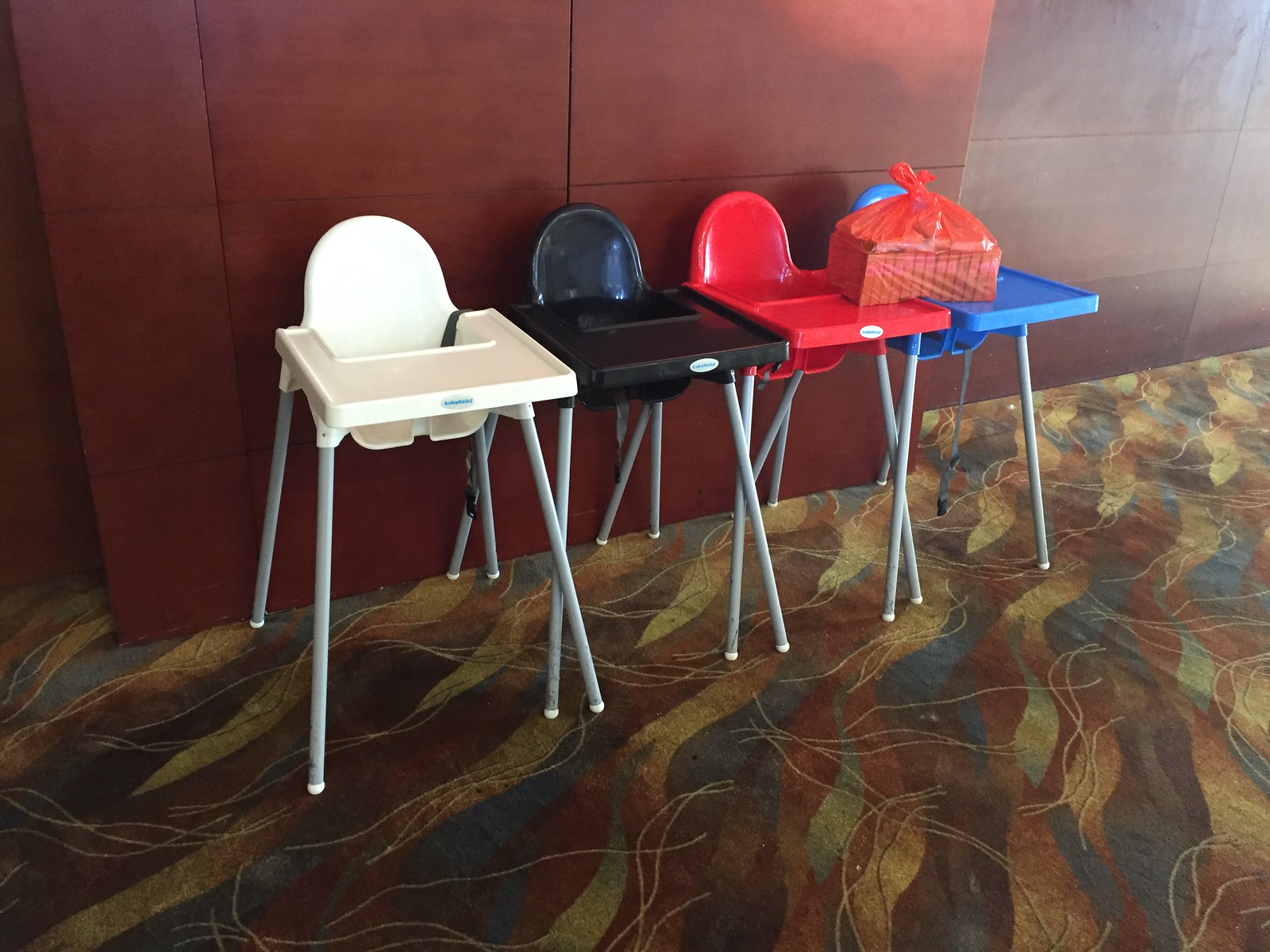This photograph features four high chairs for babies, each with four metal legs and a plastic bucket seat equipped with a seatbelt and a front tray. The high chairs are placed side by side, their legs overlapping slightly, and are identical except for their colors: white, black, red, and blue. The floor beneath them is carpeted with a pattern of blue, red, yellow, and green leaves, while the wall behind them is paneled in a reddish-brown wood divided into rectangular sections. Each high chair is closely lined up in front of the wall. Notably, a red plastic bag containing thirteen rectangular books is placed on the trays of the red and blue high chairs, with the bag tied shut.